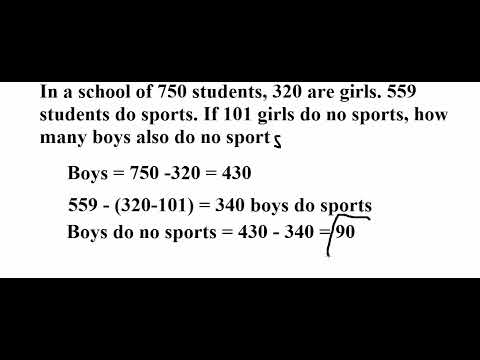The image features a black-bordered white rectangle centered between thick black bars on the top and bottom. Inside the white rectangle, bold black text presents a mathematical problem and its solution. The text reads: "In a school of 750 students, 320 are girls. 559 students do sports. If 101 girls do no sports, how many boys also do no sports?" Below this, the solution is detailed: "Boys = 750 - 320 = 430," followed by "559 - (320 - 101) = 340 boys do sports," and finally, "Boys do no sports = 430 - 340 = 90." The layout suggests this is part of a math lesson or presentation slide.